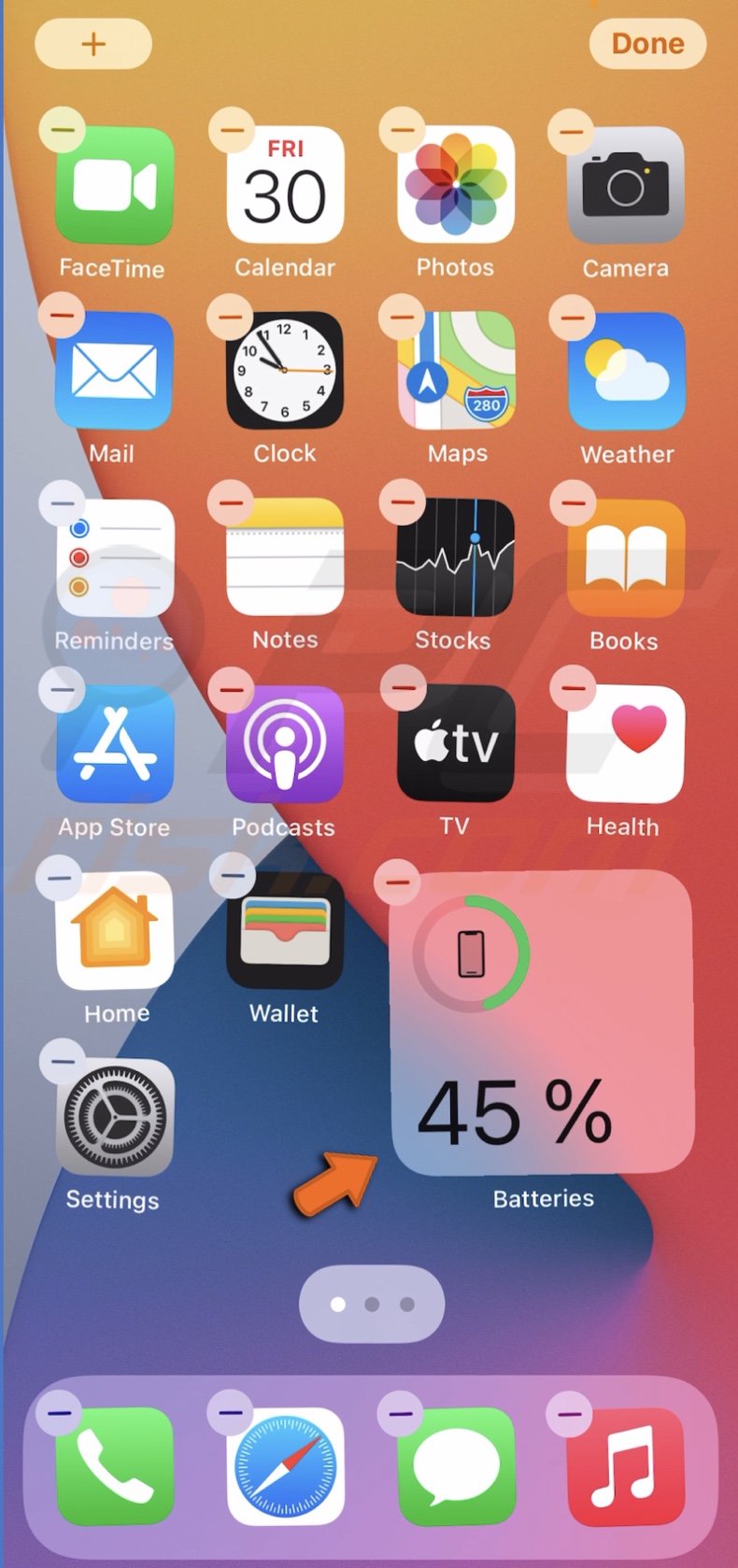This image is a detailed screenshot of an iPhone's home screen in edit mode, where icons are wiggling to indicate they can be rearranged or removed. In the upper left-hand corner of each app icon, there is a small circle with a minus sign inside, representing the option to delete the app. An orange arrow has been added to the image, pointing toward a battery widget on the screen, which shows the phone's battery level at 45%.

The iPhone is displaying a variety of apps. Starting from the top left, the apps are: FaceTime, Calendar, Photos, Camera, Mail, Clock, Maps, Weather, Reminders, Notes, Stocks, Books, App Store, Podcasts, TV, Health, Home, Wallet, and Settings. At the bottom priority bar, the user has the Phone, Safari, Messenger, and Apple Music apps pinned for quick access.

The background of the home screen features a standard wallpaper with an abstract design of orange, white, and blue circles.